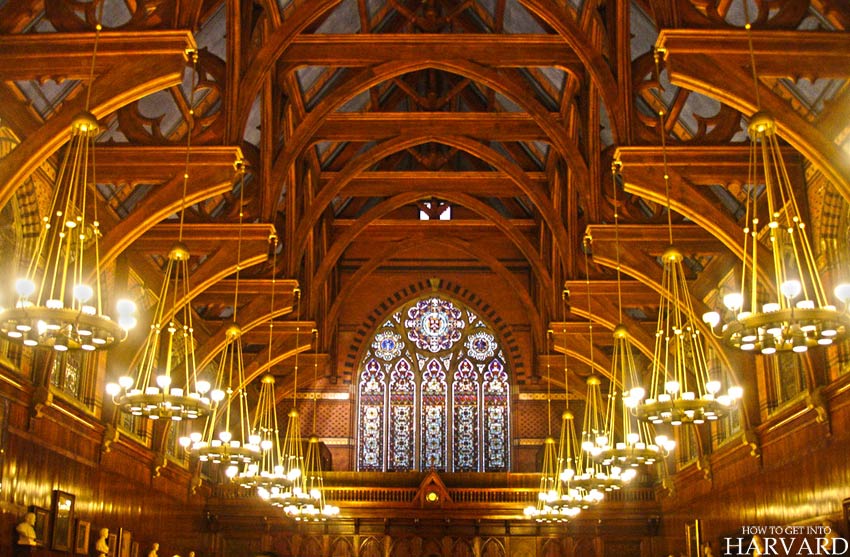The image depicts the interior of a vast and grand hall, resembling a church or a hall at Harvard University. The arched ceiling is supported by intricate wooden rafters that converge at a central point, emphasizing the height of the structure. The rafters, crafted from brown wood, have long beams extending towards the center, each adorned with curved braces and strings of lights. These lights culminate in wooden circles embedded with large, bright white bulbs, illuminating the space.

Prominently, a large stained glass window dominates the background. The window is square at the bottom and arches at the top, divided into five vertical columns. The lower section of each column features white floral patterns resembling circles. Moving upwards, there are segments of orange and purple dots, followed by purple backgrounds with white dots centered within them. Above these, a line of black dotted lines encircles the design.

Symmetrically arranged chandeliers, six on each side, hang down from the rafters, enhancing the hall’s elaborate décor with their intricate designs and bright lights. Along the sides at floor level are rows of white marble busts, adding a classical touch to the room and suggesting a setting rich in history and culture. The symmetry of the room is accentuated by these mirrored elements on both sides.

In the bottom right corner of the image, white text reads, "how to get into Harvard," hinting at a connection to Harvard University. This combination of architectural grandeur and academic reference underscores the significance and prestige of the depicted space.